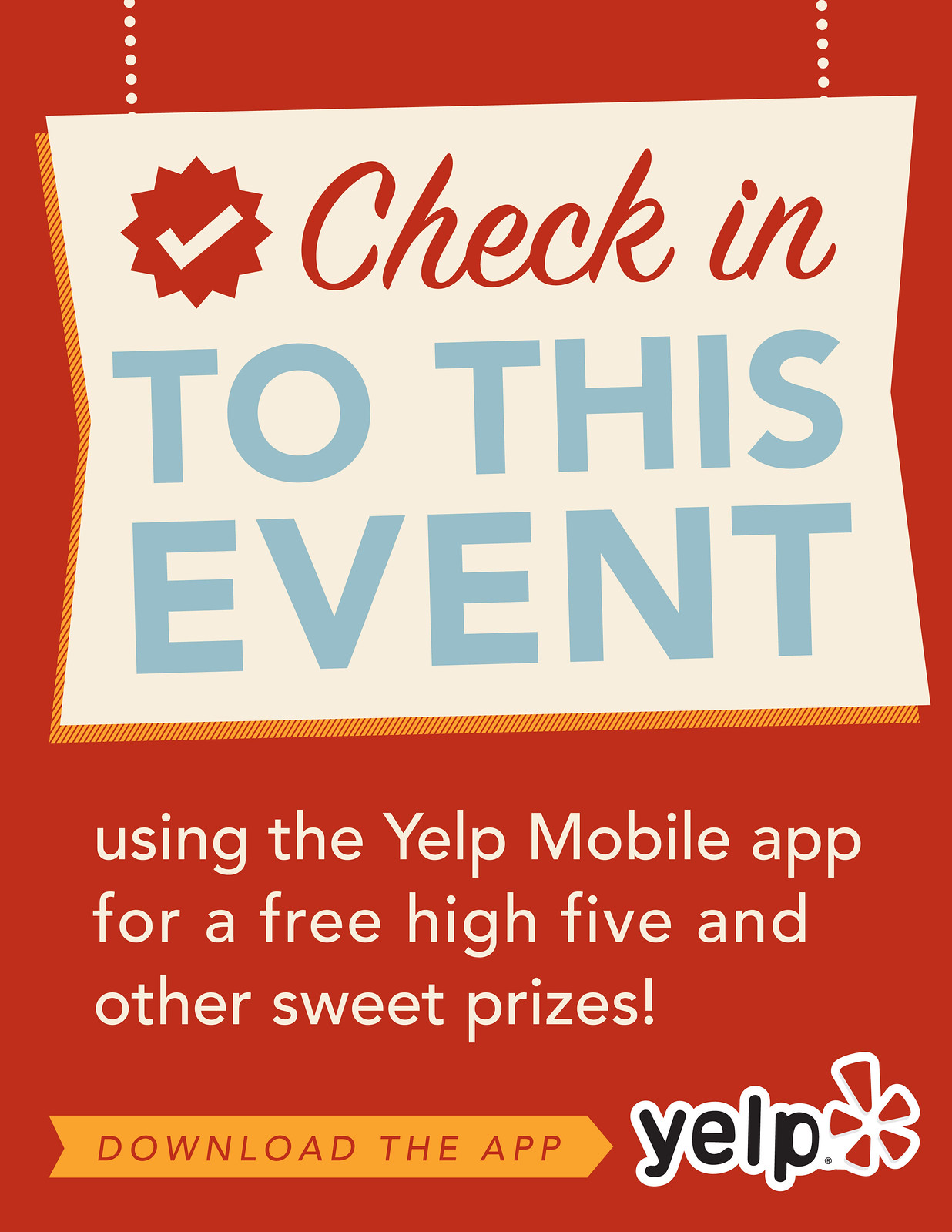The promotional banner for a review app features a vibrant red background on a rectangular shape, with the left and right sides being twice as long as the top and bottom. The image is styled to look like a sign hanging down from chains, symbolized by white dots in the top left and bottom right corners of the banner. At the top, the sign has a star with a white check mark, beside which red text reads "Check-In" and adjacent blue text says "to this event." Below this sign, white text on the red background advises users to "use the Yelp mobile app for a free high-five and other sweet prizes." A bright yellow arrow with red text instructs people to "download the app," pointing towards the Yelp logo located in the bottom right. The Yelp logo is in black text with a red symbol, both outlined in white.